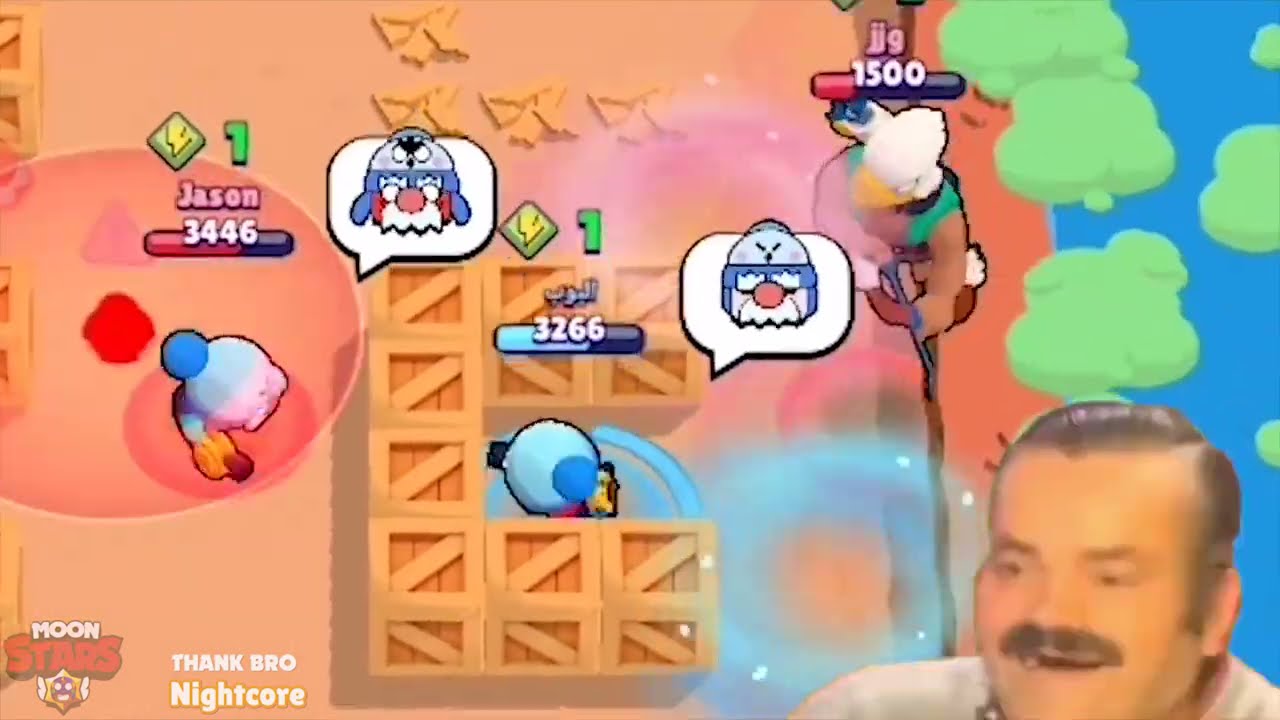The image is a low-quality screenshot from a whimsical, possibly children's video game on a mobile device or computer. The bottom left features a logo reading "Moonstars" followed by the text "Thank Bro Nightcore." Central to the image are stacked wooden crates, prominently displaying the letter "E." Various characters with health bars, including a blue-headed figure named Jason with a health score of 3,446, and another character with a score of 3,266 are visible. To the right, an armored samurai eagle labeled Jig 1500 is seen climbing, while some birds, seemingly inspired by Angry Birds, are slingshotting through the air. The background includes vibrant hues of red, pink, brown, light blue, and green. In the bottom right corner, there is a meme of the Keck W guy, partially showing his head and shoulders, with green clouds above him against a blue background, suggesting thoughts or ideas. The entire scene is set against a light beige background with brown elements scattered throughout, creating an overall playful and colorful atmosphere.